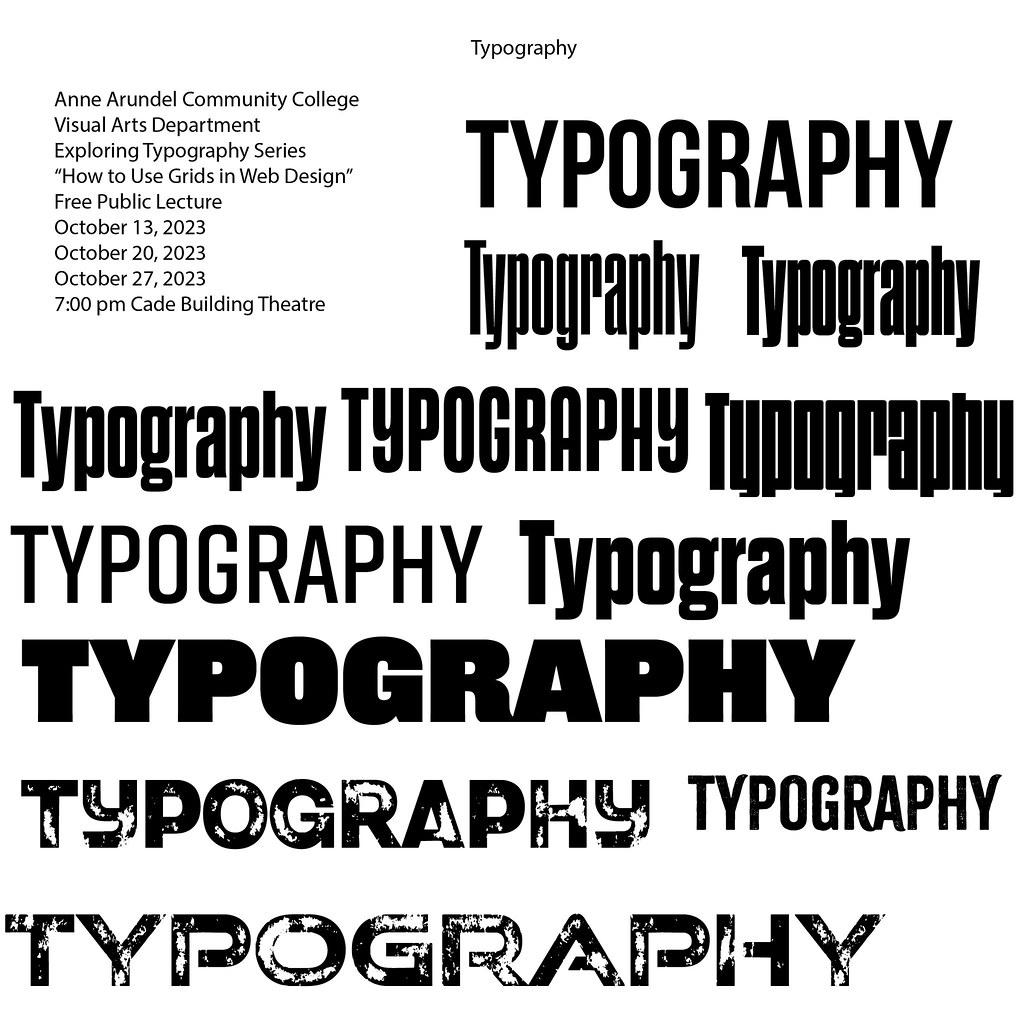The image has a clean white background with black text. In the top left corner, it reads: "Anne Arundel Community College, Visual Arts Department, Exploring Typography Series, How to Use Grids in Web Design, Free Public Lecture, October 13, 2023, October 20, 2023, October 27, 2023, 7 p.m., Cade Building Theater." Below this detailed information, the word "Typography" is repeatedly written in various fonts and sizes, arranged in several lines filling the rest of the image, showcasing an assortment of typographic styles.